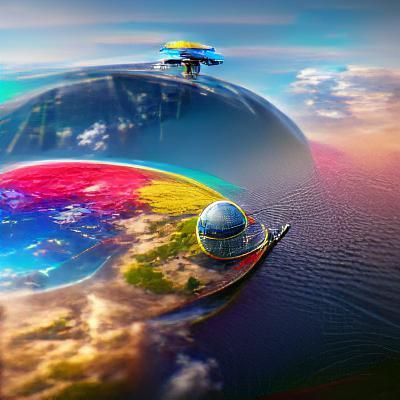This artwork is an abstract, futuristic animation that vividly merges sky and ocean in a surreal landscape. The sky boasts a gradient of bright teal, blue, and white clouds, transitioning to sunset hues of orange and pink and blending into the dark blue ocean below. In the distance, there's a vivid blue sky with scattered clouds enhancing the scenery's ethereal quality. The left side features a large, dark blue dome adorned with yellow and blue accents, positioned near land that is a blur of brown and green tones, marked with patches of bright yellow, pink, and blue vegetation alongside some seemingly dead, brown areas. A shiny, circular silver structure stands centrally amidst this colorful terrain, while another, more pronounced chrome-like blob sits at the tip. These two highly futuristic, sci-fi structures - one between what seems to be an ocean and a lake and the other atop a possible hill or mountain - are unlike anything seen on Earth today.